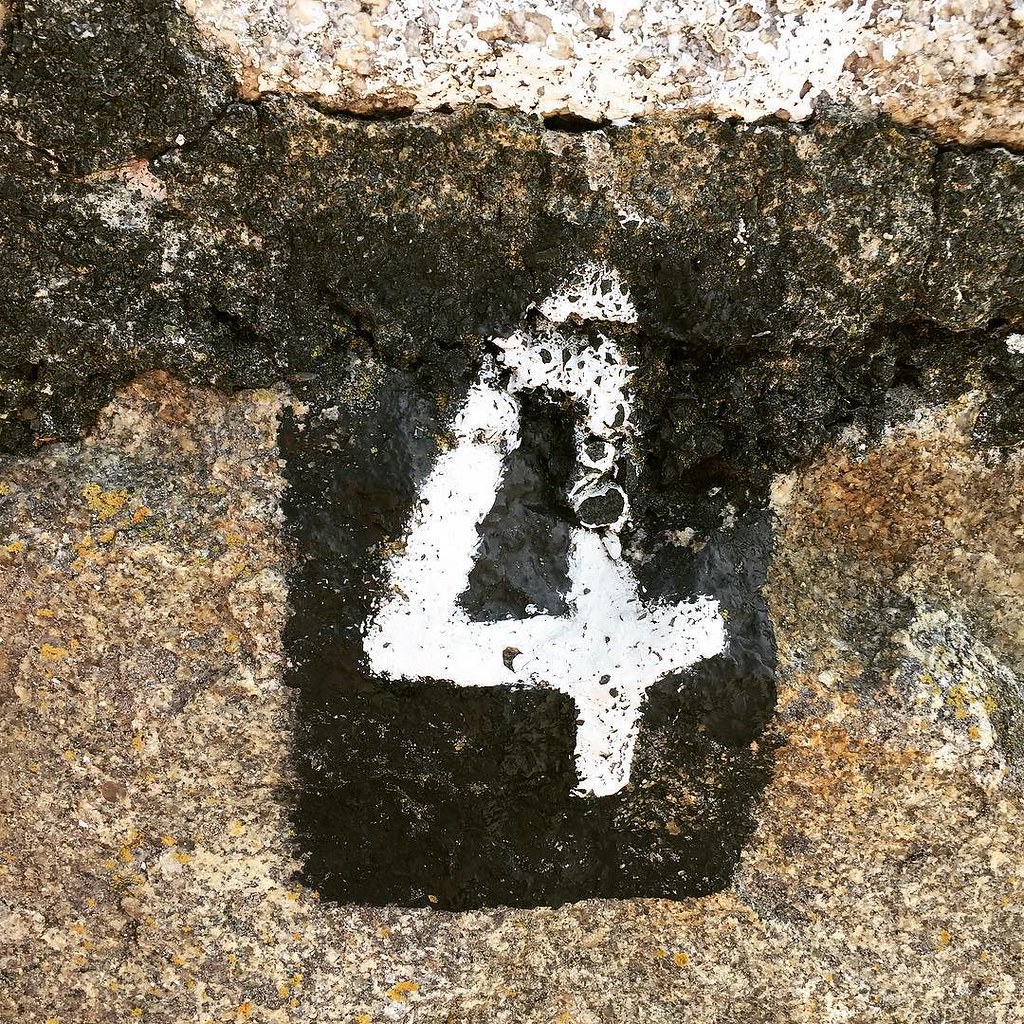The photograph depicts a close-up of a multi-colored stone wall, featuring a prominent black rectangular area in the center with a large white number "4" spray-painted on it. The wall comprises various hues, including cream, orange, brown, white, and black, suggesting either natural stone or granite. At the top of the image, there is an inch or two of stone that transitions into the central black rectangle. This painted section occupies the middle of the image, clearly contrasting with the surrounding stones. The stones themselves vary in color, from quite dark shades at the bottom, more brownish hues in the middle, to lighter, almost white tones at the top. The image has a bright, outdoor feel, though no other contextual details about the setting or structure of the wall are visible.